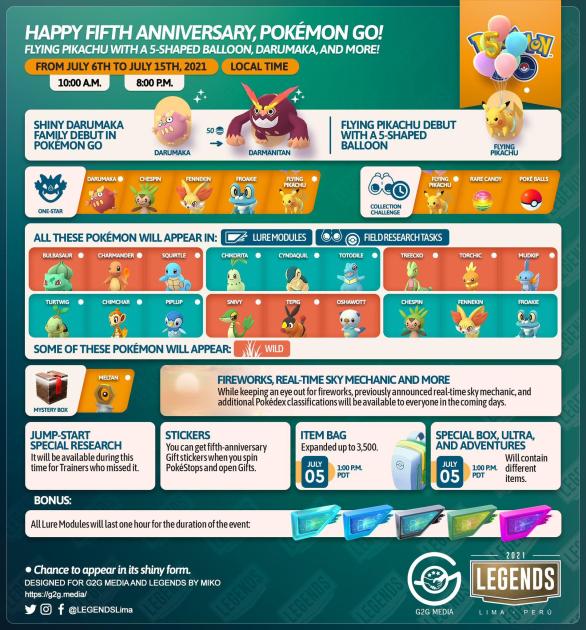In celebration of Pokémon GO's 5th Anniversary, an ad features a vibrant image capturing key event details and characters. At the top, bold text reads "Happy 5th Anniversary, Pokémon GO," setting a festive tone. The image highlights special Pokémon appearances such as Flying Pikachu with a "5"-shaped balloon and Shiny Darumaka, alongside other anticipated debuts.

The event spans from July 6th to July 15th, 2021, running daily from 10 a.m. to 8 p.m. local time. Underneath this schedule, it emphasizes the debut of the Shiny Darumaka family and Flying Pikachu with a unique "S"-shaped balloon.

A "Collection Challenge" section is noted, adjacent to a pair of binoculars, indicating that various Pokémon can be encountered through lure modules and field research tasks. The Pokémon list is organized into color-coded sections: three highlighted in orange, followed by three in teal, another set of three in orange, a row with teal, then orange, and ending with teal.

Subsections below list specific areas for increased chances of encountering Shiny forms of certain Pokémon, adding another layer of excitement for players. The ad is visually engaging and rich with detailed instructions, ensuring that fans are well-informed about the event's exciting features.